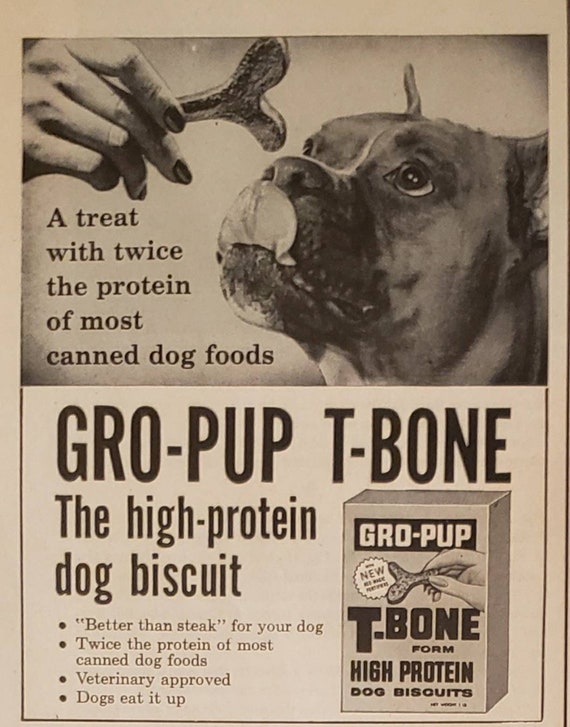A sepia-toned, black and white advertisement, likely from an old magazine or newspaper, for GrowPup T-Bone High-Protein Dog Biscuits. The top half of the ad features an intricately detailed illustration of a woman’s manicured hand holding a bone-shaped treat, extended towards a boxer dog with a brown face and distinct white markings. The dog is licking its lips in eager anticipation. This section includes the text, "A treat with twice the protein of most canned dog foods.” Below this image, the ad showcases a box of GrowPup T-Bone biscuits, alongside a bullet-pointed list highlighting the product’s benefits: "Better than steak for your dog," "Twice the protein of most canned foods," "Veterinary approved," and "Dogs eat it up." The entire layout exudes a vintage charm, enhanced by the aged, yellowed appearance of the advertisement’s paper.